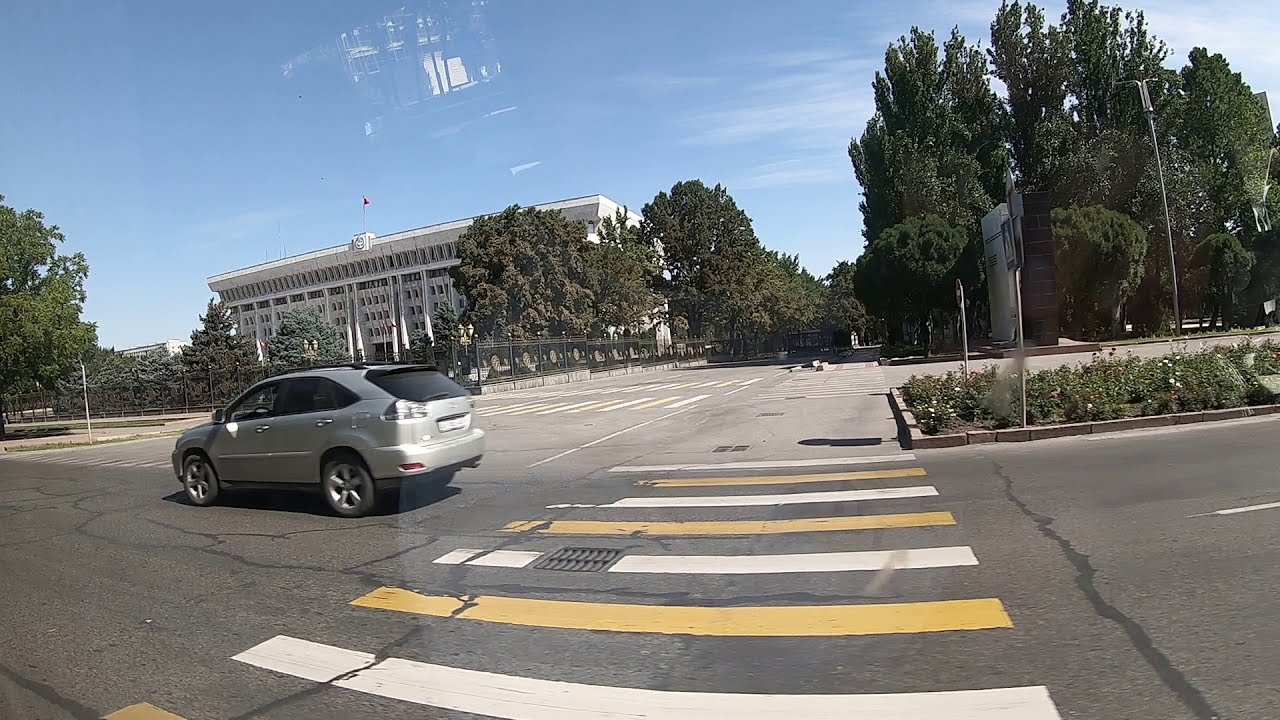This detailed daylight photograph captures a bustling road scene, seemingly taken from within a vehicle, indicated by the faint glass reflections in the center. The viewer looks across a multi-lane asphalt street from the curb, with a prominent pedestrian crosswalk marked in yellow and white stripes. 

To the left, a silver SUV with tinted windows has recently passed the walkway. The street splits into two lanes each way, divided by a median adorned with green plants and low flowers. On the right side of the median is a brick curb. Additional signage on the median is present, but not legible from this angle. 

Lush, tall green trees line both sides of the road, with a lamppost visible on the right. In the far background to the left stands a massive, multi-story white building with brutalist architecture, characterized by its many windows and stark concrete facade. Atop this building flutters a red flag against the blue sky, which is dotted with thin, wispy white clouds. The overall setting is clearly outdoors, with pleasant weather enhancing the scene.